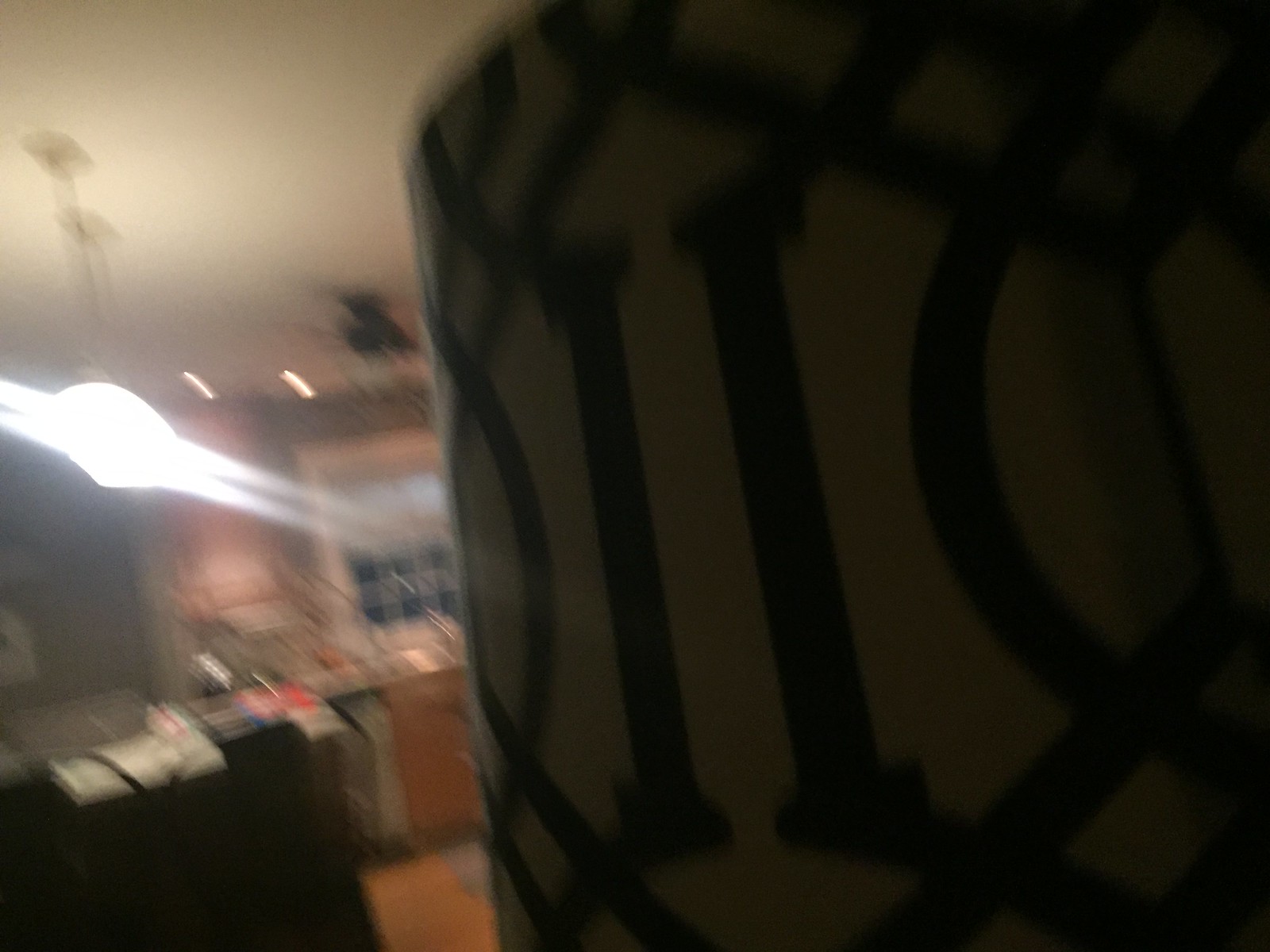This blurry, out-of-focus photograph captures a chaotic, yet intriguing scene in a domestic setting. On the left side, an illuminated room can be partially seen, possibly a kitchen, with a bright white light emanating from the ceiling. The light appears to have rings around it, resembling a planet, which is a result of the camera shutter speed distorting the image. Above the glowing orb are two pendant lights, visibly wired into the ceiling, though the light fixtures themselves are obscured by the blinding brightness.

Within this room, a window is visible above some cabinetry, suggesting the presence of a sink directly below it. Lower cabinets are discernible, as well as a hint of a hardwood floor with a brownish hue. In the lower left corner of the foreground, there is a black and red object that seems to be made of plastic or metal, possibly a camera, though its exact nature remains uncertain due to the image's quality.

On the right side of the photo, a close-up view reveals a drum-shaped object that could be a lampshade. It appears to be linen-colored with intertwining blue and brown designs. A Roman numeral "II" is prominent on the front, surrounded by more intricate patterns. The exact identity of this item remains ambiguous; it could equally be a table with a decorative tablecloth.

Overall, the photograph offers a tantalizing glimpse into a cluttered and visually stimulating environment, capturing an interplay of light, color, and form.